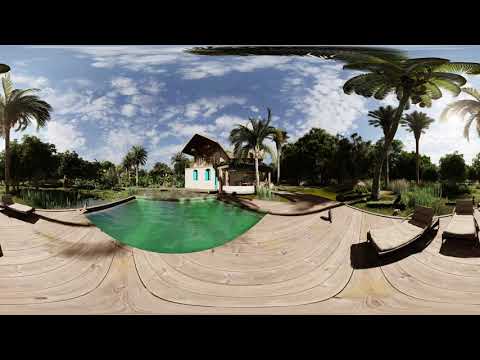This panoramic 360-degree photograph vividly captures an outdoor tropical oasis featuring the backyard of a white house with blue windows, prominently showcasing a turquoise-green, half-circle pool slightly off-center towards the left. Surrounding the clear pool, the wooden plank walkway seamlessly merges into a natural-colored deck area adorned with three lounge chairs for relaxing. The tropical ambiance is heightened by several palm trees interspersed amidst various other types of trees and lush greenery, set against a vibrant blue sky filled with scattered thin white clouds. To the left of the pool, a serene body of water, likely a pond or lake, complements the scene, further enhancing the tranquil and lush environment that surrounds the backyard retreat.